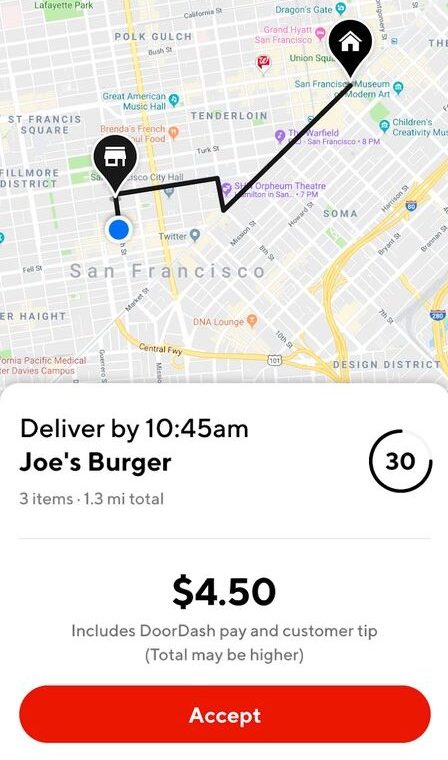A detailed screenshot from the DoorDash app for drivers shows a map centered around San Francisco. The map prominently displays various neighborhoods and landmarks such as the Tenderloin, Soma, San Francisco Museum of Modern Art, Dragon's Gate, Grand Hyatt San Francisco, Polk Gulch, Lafayette Park, St. Francis Square, Fillmore District, and Design District. Highlighted on the map is a marked delivery route. An overlay at the bottom of the screen instructs the driver to deliver by 10:45 a.m. an order from Joe's Burger consisting of three items totaling 1.3 miles. To the right, a partially-obscured circle displays the earnings as $4.50, which includes DoorDash pay and customer tip, with a note indicating the total may be higher. A red button with the word "accept" in white letters is prominently displayed, inviting the driver to take the order. The screenshot lacks any photographic elements, and there are no people, animals, birds, plants, or trees shown.